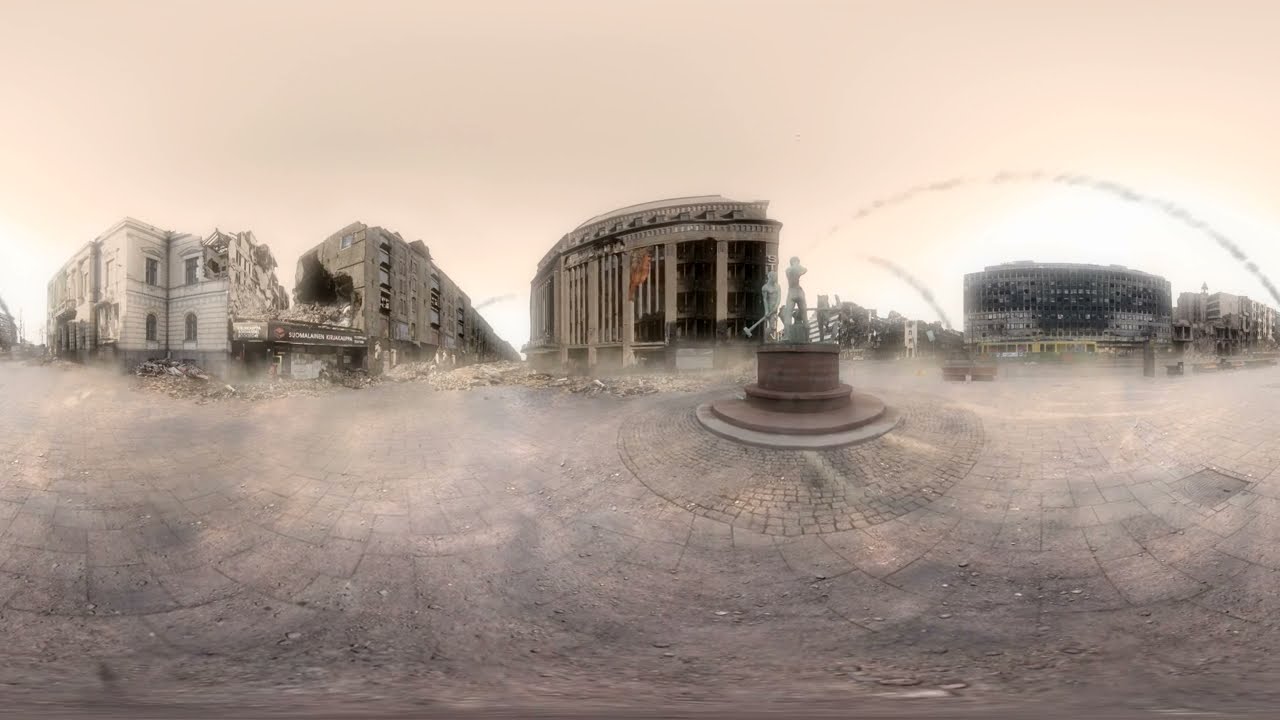The image showcases a dreary, war-torn cityscape under a peach-colored, cloudy sky. At the center, slightly to the right, stands a prominent statue of two workers wielding sledgehammers, raised on a brown pedestal amidst a broad, stone-paved city square. Surrounding this central feature are various buildings in different states of disrepair. To the left, there's a mostly intact yet slightly burned building with a flag, juxtaposed against other structures marred by bombing, with a particularly notable building sporting a large gaping hole. On the right, additional buildings appear to be burned and heavily damaged, contributing to an overall scene of devastation and rubble. The entire location suggests a city that has endured significant hardship, its somber tones of tan, brown, gray, and muted light blue augmenting the sense of abandonment and despair. A billboard is visible, although its text is indiscernible. Additionally, the image is designed with a "bubble effect," giving it a slight curvature, implying it can be wrapped into a cylindrical form to form a continuous panoramic view.